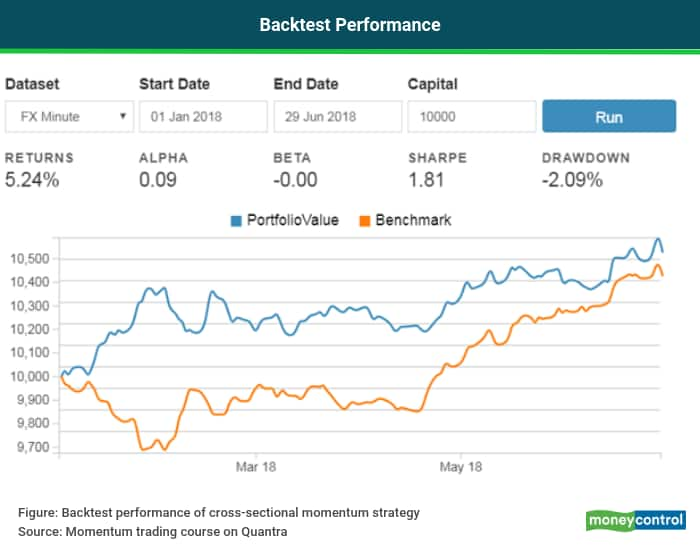This image features a detailed depiction of a backtest performance screen for financial data analysis. At the top, there is a greenish-blue header labeled "Back Test Performance." Directly below this header is a horizontal green line, approximately an eighth of an inch thick. The main section of the interface features various input fields, including drop-down boxes for selecting the data set, start date, end date, and initial capital. To the right of these boxes is a blue "Run" button.

Beneath these input fields, a summary of key performance metrics is displayed: Returns at 5.24%, Alpha at 0.9%, Beta at 0, Sharpe Ratio at 1.81, and a Drawdown at -2.09%. Below this summary, two colored squares—blue for Portfolio Value and orange for Benchmark—provide a legend for the graph beneath them.

The graph charts the performance from March 18th to May 18th, with values ranging from 9,700 to 10,500. The blue line representing the portfolio value shows relative consistence with a peak near 10,500. Conversely, the orange benchmark line dips initially before fluctuating and finishing at nearly 10,400 by the end of May. The image encapsulates a period of stable portfolio performance compared to a more volatile benchmark trajectory.